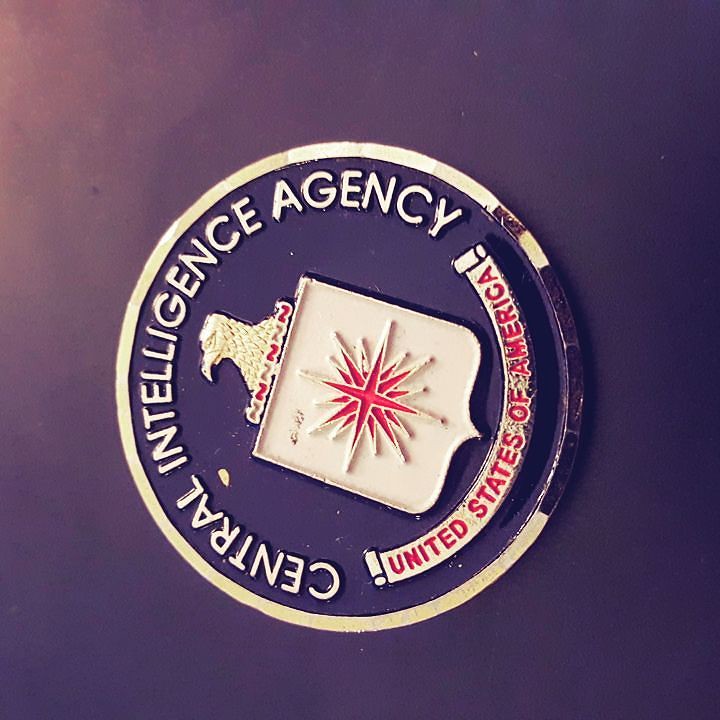The image depicts an aged and possibly worn Central Intelligence Agency insignia. The emblem is centered within a reflective silver or gray circle, which shows signs of tarnish, revealing patches of blue. The background is a deep, dark blue or very dark purple, appearing almost metallic. Across the top arc of the circle, in silver capital letters, reads "Central Intelligence Agency." Below this, in the bottom portion, a silver banner with red text spells out "United States of America."

At the center of the insignia is a distinct shield, featuring a red starburst pattern. An eagle, facing left from the viewer’s perspective, is perched atop the shield. Between the eagle and the shield, white and red wavy lines add to the intricate design. The emblem appears to be slightly tilted to the left, suggesting it is either stamped on a surface or part of a collectible coin. The repeated motifs and the overall design imply a sense of historic wear, giving it a vintage appeal rather than a new, unblemished appearance.